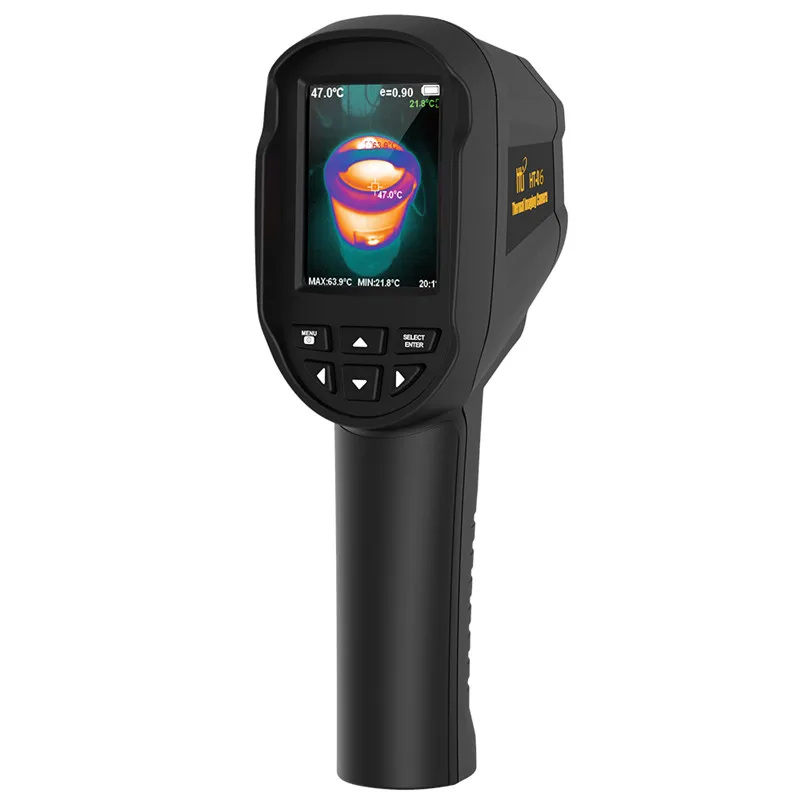This image features a handheld black instrument resembling a thermometer gun, shown from a front point of view, allowing a clear view of its screen and buttons. Central to the screen is a thermal image displaying a colored representation with yellow, orange, blue, and purple hues, indicating thermal energy. The screen also shows critical measurements: the temperature reads 47.0 degrees Celsius, the emissivity ('E=0.90') is noted on the top left, and there are max and min temperature readings of 63.9 degrees Celsius and 21.8 degrees Celsius, respectively. The battery icon on the top right indicates full battery life. Below the screen, there are six clearly labeled buttons arranged in two rows of three: Menu, Up, Down, Left, Right, and Select/Enter. The device also displays additional readings such as '20°F' on the bottom right. It features a black and yellow brand logo on the right-hand side. The instrument has a model number HT-16, suggesting its use for precise thermal measurement.